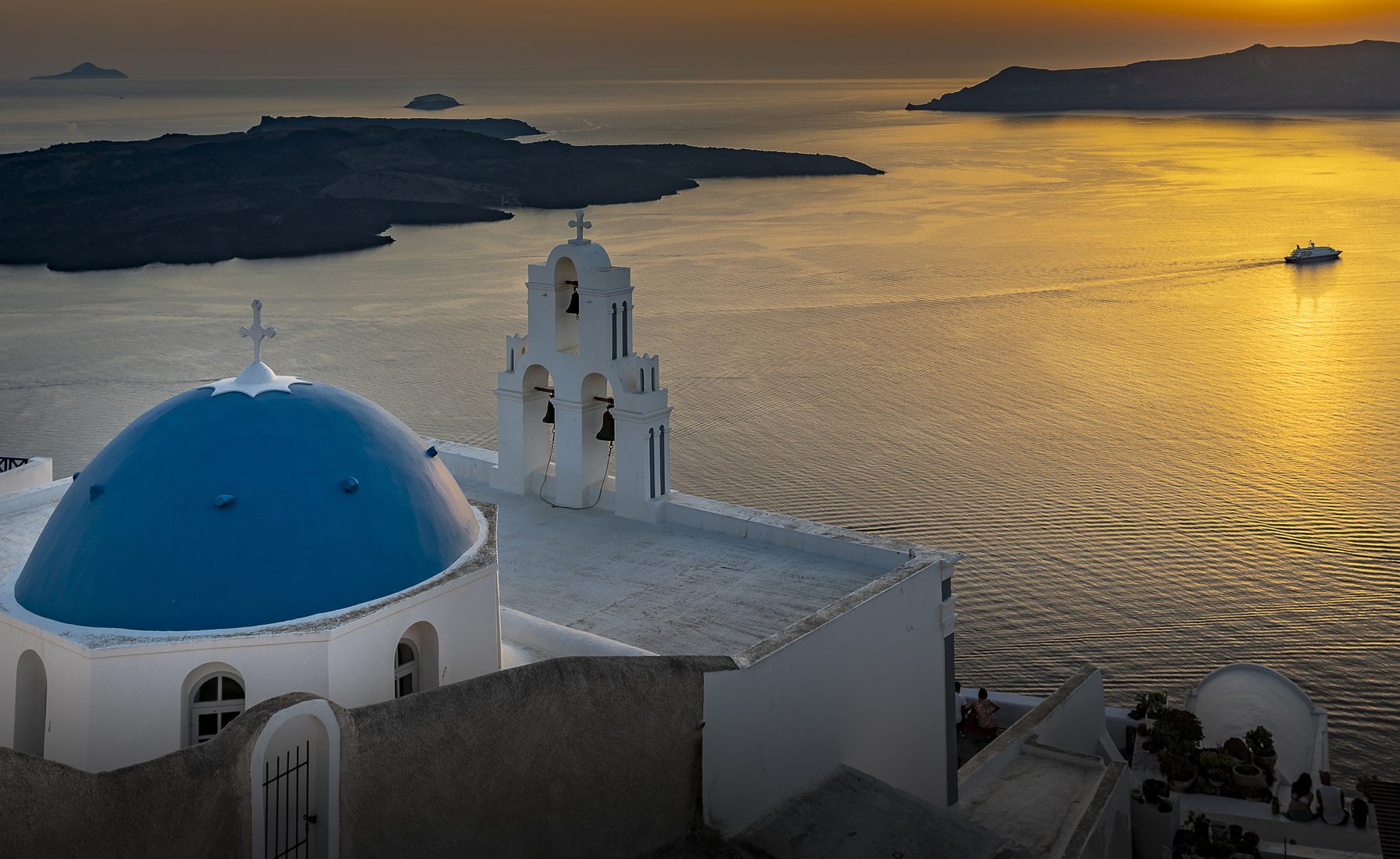This elevated photograph captures a picturesque scene likely set on a Greek island, with emphasis on a beautiful, white church adorned with a large blue dome crowned by a white cross. The church's distinctive architecture also includes a clock tower and a bell tower comprising three bells arranged in a triangle, each held within arched supports topped by another cross. The vantage point offers a breathtaking view of the ocean below, which glimmers in shades of gold and orange from the setting sun, visible just out of frame to the right. Strikingly visible are several small islands silhouetted against the warm-hued water; one island is seen on the top right, another towards the left, and a third one far off in the top left corner. Enhancing the serene seascape, a cruise ship sails in the distance, while a smaller boat is more centrally placed in the radiant waters. The setting sun casts a gradient in the sky, transitioning from bright orange on the right to a softer, duller hue towards the left, completing this idyllic maritime scene.